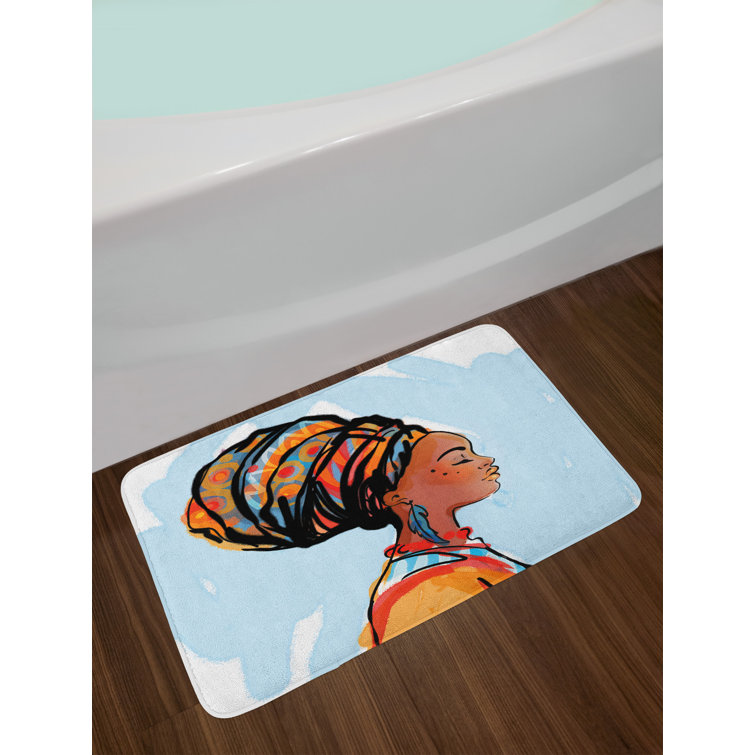The image is a color photograph showcasing a bath mat prominently displayed on a dark wooden or wood-like floor next to a white, molded acrylic bathtub filled with slightly aqua-colored water. The bath mat, which has a low cushiony texture and rounded corners, features a vivid, watercolor-like design. The central figure on the mat is an African-American woman in profile, facing right. She is adorned with a vibrant turban wrapped around her head, which is edged in black and showcases a palette of bright blues, oranges, reds, and a touch of white. She wears striking long blue feather earrings and a red necklace. Her eyes are closed, and she has three dots on her cheekbone. The attire she wears has matching colorful patterns, incorporating blue and white stripes, and hues of red and orange. The background of the mat is a light blue watercolor wash over a white base, adding a soft yet contrasting backdrop to the bold, colorful figure.